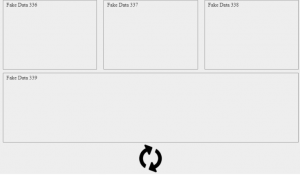Screenshot of a wireframe layout displaying an empty grey page with placeholder elements. At the top, there are three evenly sized and spaced boxes, each outlined with a thin grey line and featuring small checkmarks in their upper left corners. Below these, there is a longer, empty rectangular box that spans the entire width of the page. Beneath this rectangle, a black refresh icon is positioned centrally. The area below this icon consists of an empty space, providing room for additional content or elements.